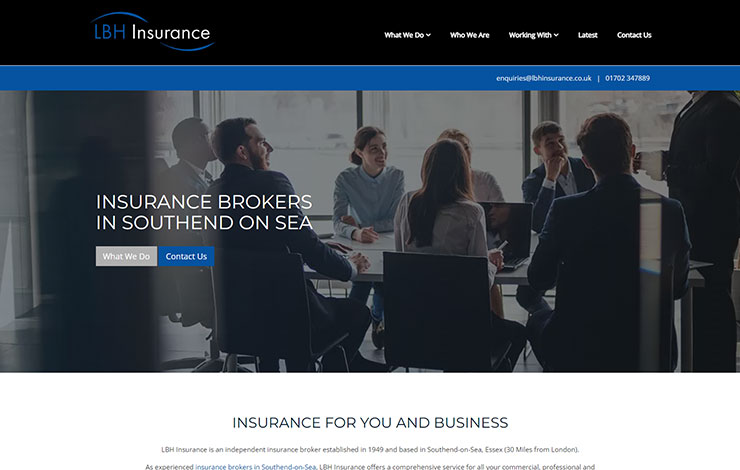The image displays the screen for LBH Insurance's website. The logo prominently features "LBH" in blue, with "Insurance" in white. Above the "LBH" letters, there is a design element resembling an eyebrow in blue that starts at the letter "L" and arcs over to the end of the word "Insurance," creating a sense of motion or flow. Below this blue arc is a complementary element, resembling an upside-down eyebrow, giving the logo a three-dimensional appearance.

Below the logo, text reads "Insurance Brokers in Self and on C," accompanied by options such as "What We Do" and "Contact Us." There is also a tagline emphasizing "Insurance for You and Business."

The main visual on the screen is a wide-angle photograph of a professional meeting. A group of male and female staff members are seated around a large table, attentively looking at a speaker standing to the right. The men are dressed in suits, while the women wear professional attire, all appearing engaged and pleased with the speaker's presentation.